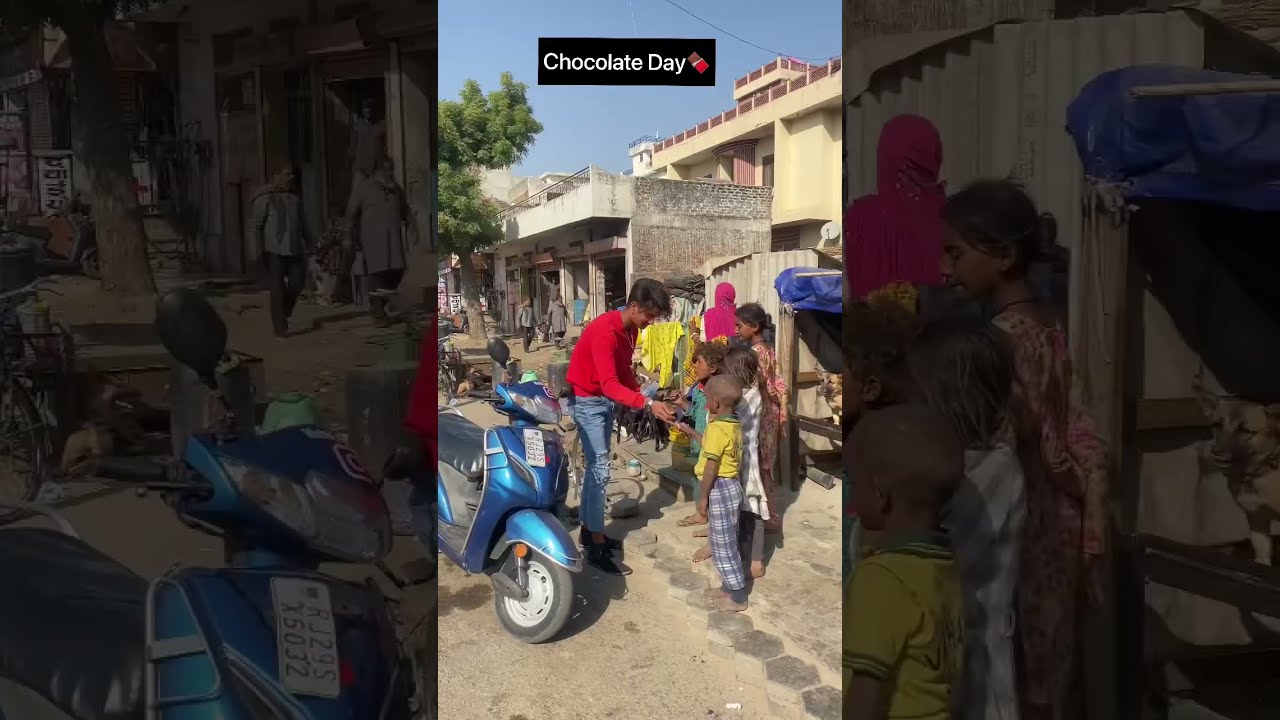The image is segmented into three vertical sections, with the first and third sections displaying darkened close-ups of the central section. The central section depicts a scene that appears to take place in a rural Indian village. Here, a young Indian man, with no facial hair and black hair, is seen wearing a red long-sleeve t-shirt and blue jeans. He is standing next to a blue Vespa scooter, parked on the left side of the frame on a paved, cobblestone-style road. The man is interacting with a group of children and possibly an older girl or woman, who appear to be in worn, colorful clothing. He seems to be offering something, likely money or chocolate, as the children, who have dark skin and seem to come from a poorer background, gather around him. In the background, there are several plain-looking rectangular cement buildings varying in height, and a tree is visible towards the top left of the image. The sky above is clear and blue. A black rectangular text box with white letters at the top of the image reads "Chocolate Day," accompanied by a chocolate bar emoji. Additionally, there is an overhead wire visible in the sky.